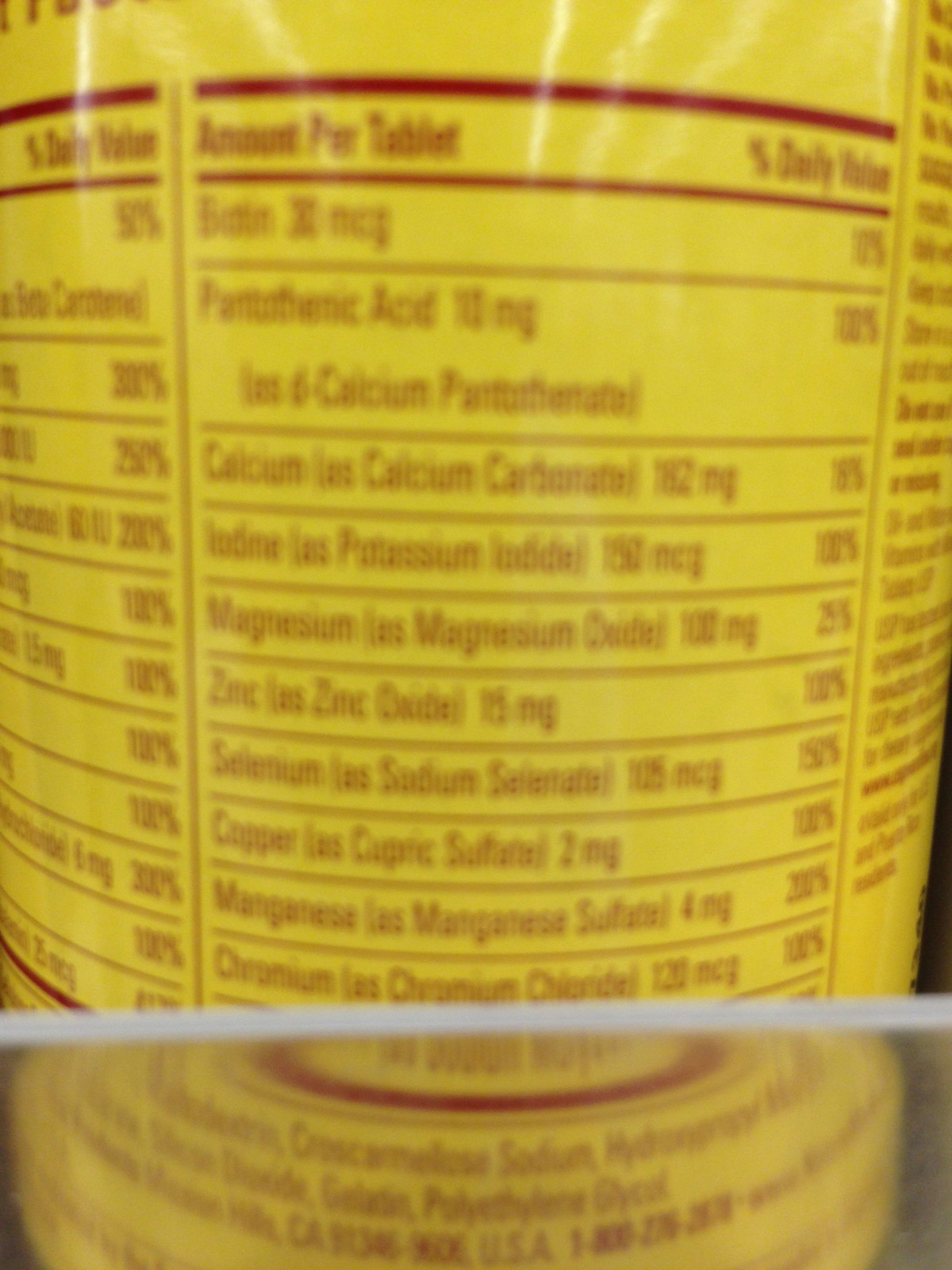This is a photograph of the nutritional facts label on what appears to be a supplement bottle. The yellow packaging is prominently featured, with the nutritional information presented in deep red text. The label, though blurry and somewhat out of focus, lists the amounts per tablet and the percentage of daily values, including a variety of vitamins and minerals like biotin, pantothenic acid at 10 milligrams, calcium carbonate at 162 milligrams, magnesium, zinc, selenium, copper, manganese, and chromium. Below the primary list, a horizontal white line seems to magnify ingredients such as sodium, gelatin, and polyethylene glycol. The label also includes details indicating it was made in California, with a visible 1-800 phone number for customer inquiries.